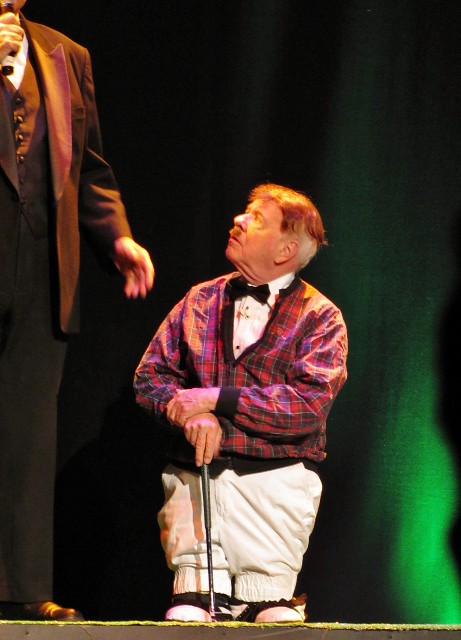In this image, two men, likely from a stage performance, are depicted under dramatic green and dark lighting. The man on the left, resembling an actor from the Carol Burnett Show, stands full-sized in a brown sports jacket, matching vest, and brown pants, holding a microphone. The man on the right, who appears significantly shorter due to clever costume alterations, is likely Tim Conway. Dressed in a red and purple plaid jacket, white undershirt, white pants, black bowtie, and tennis shoes, he wears a small red wig and mustache. Conway is looking up humorously at his taller companion while holding a golf club, leaning on it with both hands. The backdrop transitions from dark on the left to greener hues on the right, adding to the dramatic stage setting.